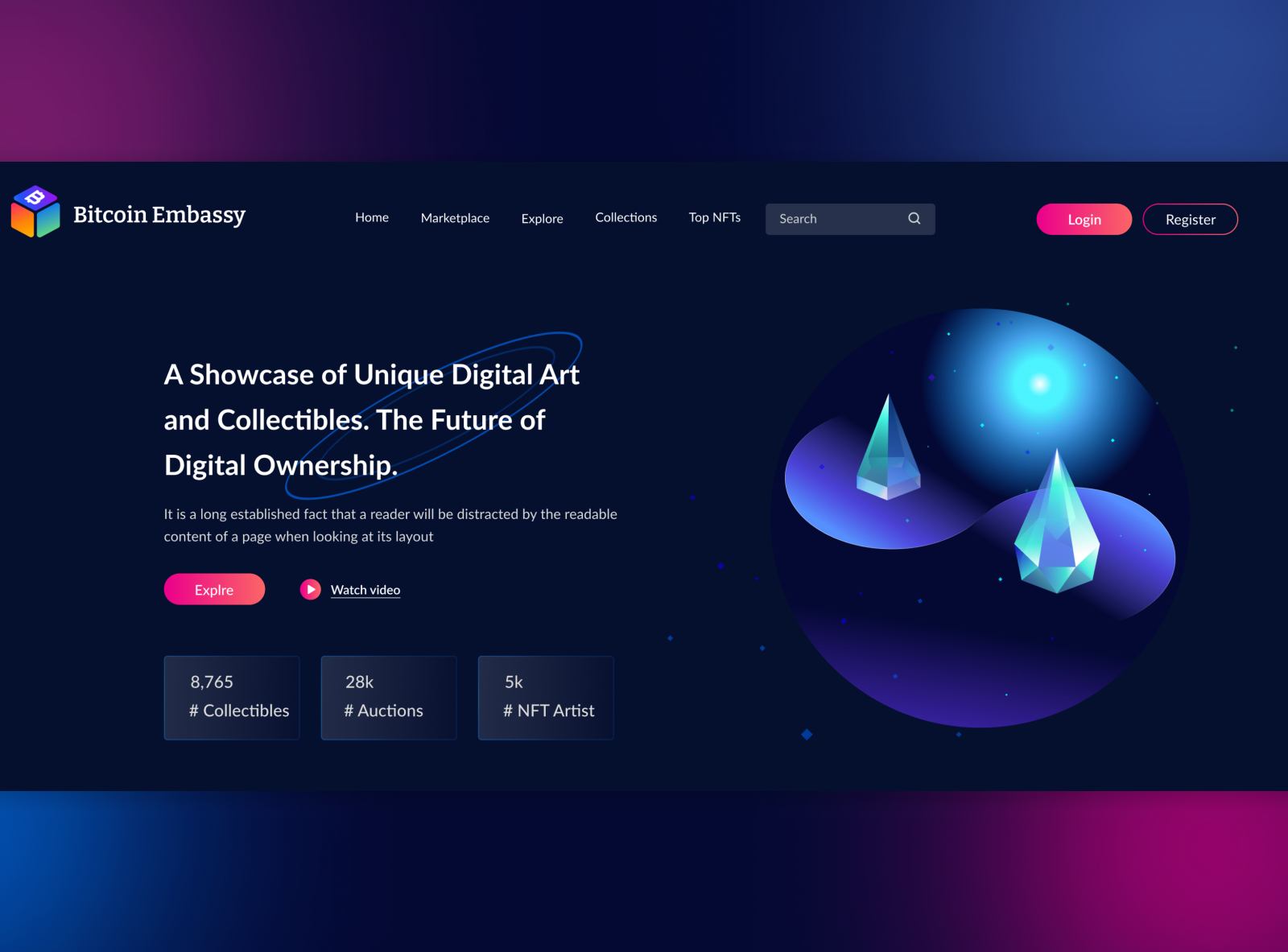The screenshot captures the homepage of the Bitcoin Embassy website, immersed in a palette of dark, swirling purple and black hues at the very top without any overlaid text. 

On the left side of the page, there is an image of a tri-sided die featuring the letter "B" on one of its faces, right next to the text "Bitcoin Embassy." 

Spanning across the screen, in small white text, are navigation links labeled "Home," "Marketplace," "Explorer," "Collections," and "Top NFTs." Adjacent to these links on the right side is a search bar with the placeholder text "Search," followed by "Login" and "Register" buttons.

Dominating the right portion of the page, a main image depicts a futuristic, outer space scene complete with sparkling stars and a night sky, showcasing several large, sharp-pointed diamond-like structures.

To the left of this image, in the largest and most prominent white text on the page, is the headline: "A Showcase of Unique Digital Art and Collectibles, The Future of Digital Ownership." Below this, a smaller text block states, "It is a long-established fact that a reader will be distracted by the readable content of a page when looking at its layout." 

To the left, a button labeled "Expire" and a "Watch Video" play button are prominently displayed. Beneath this area, three informative boxes present quick statistics: the first box states "8,765 #collectibles," the second reads "28k #auctions," and the final box says "5k #NFTartists."